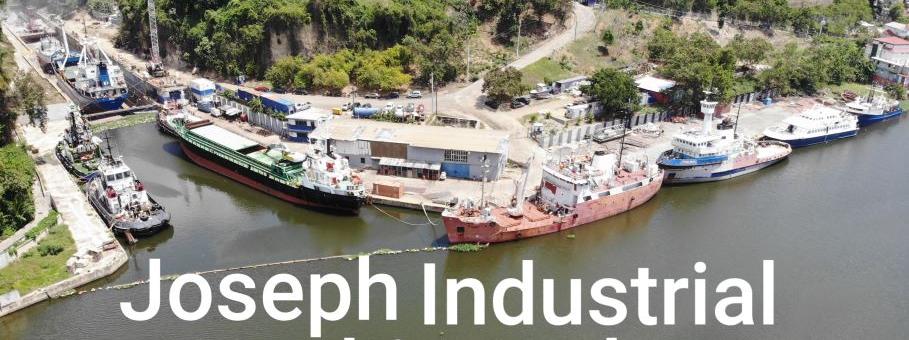An aerial, horizontal photograph, likely captured by a drone, depicts a bustling marina labeled with bold white text "Joseph Industrial" at the bottom. The image centers around a waterway populated with about eight or nine long cargo boats, most of which appear to be empty, positioned near a dock alongside a stretch of land. The dock area boasts multiple warehouse-like buildings and a walkway adjacent to the boats. Notable vessels include a large brown and white boat angled towards the right corner of the image, a distinct pink boat with a white top, and a sleek white boat featuring a blue deck. Behind these structures, a road runs parallel to the water, eventually curving upwards around a densely wooded cliff. Heavy machinery, possibly cranes, can be spotted on a dirt road in the background, adding an industrial touch to the otherwise serene, muted-colored landscape.